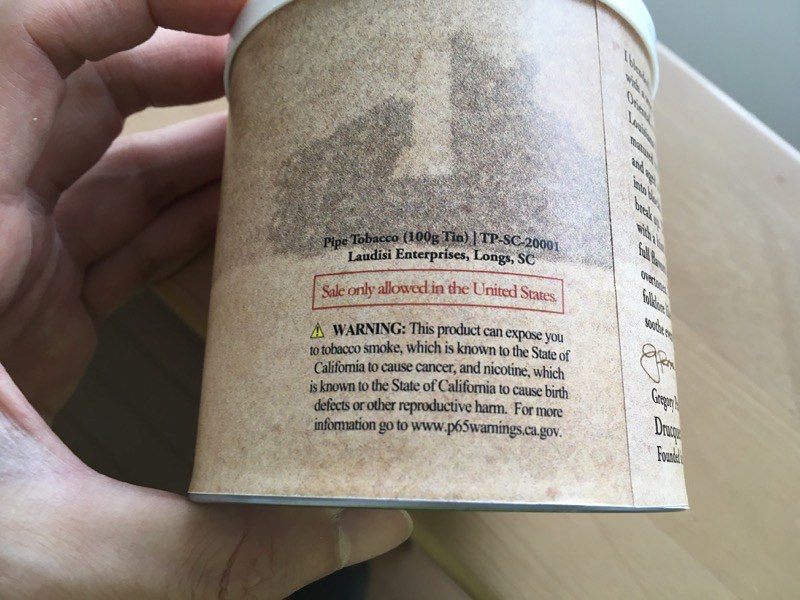This is a detailed close-up photograph of someone holding a small, light brown canister in their hands. The rectangular image, captured in landscape view, features a 100-gram tin of pipe tobacco. Prominently displayed near the top of the canister are the words "Pipe Tobacco" in bold lettering. Below this, a red box with white text stipulates "Sale only allowed in the United States." Just beneath, there is a California state disclosure warning highlighted by a yellow triangle with an exclamation point. The scene is set against a backdrop of light brown wood, adding a rustic element to the image and complementing the canister's earthy tones. The person's hands firmly grasp the tin, emphasizing the intimate, tactile nature of the moment.